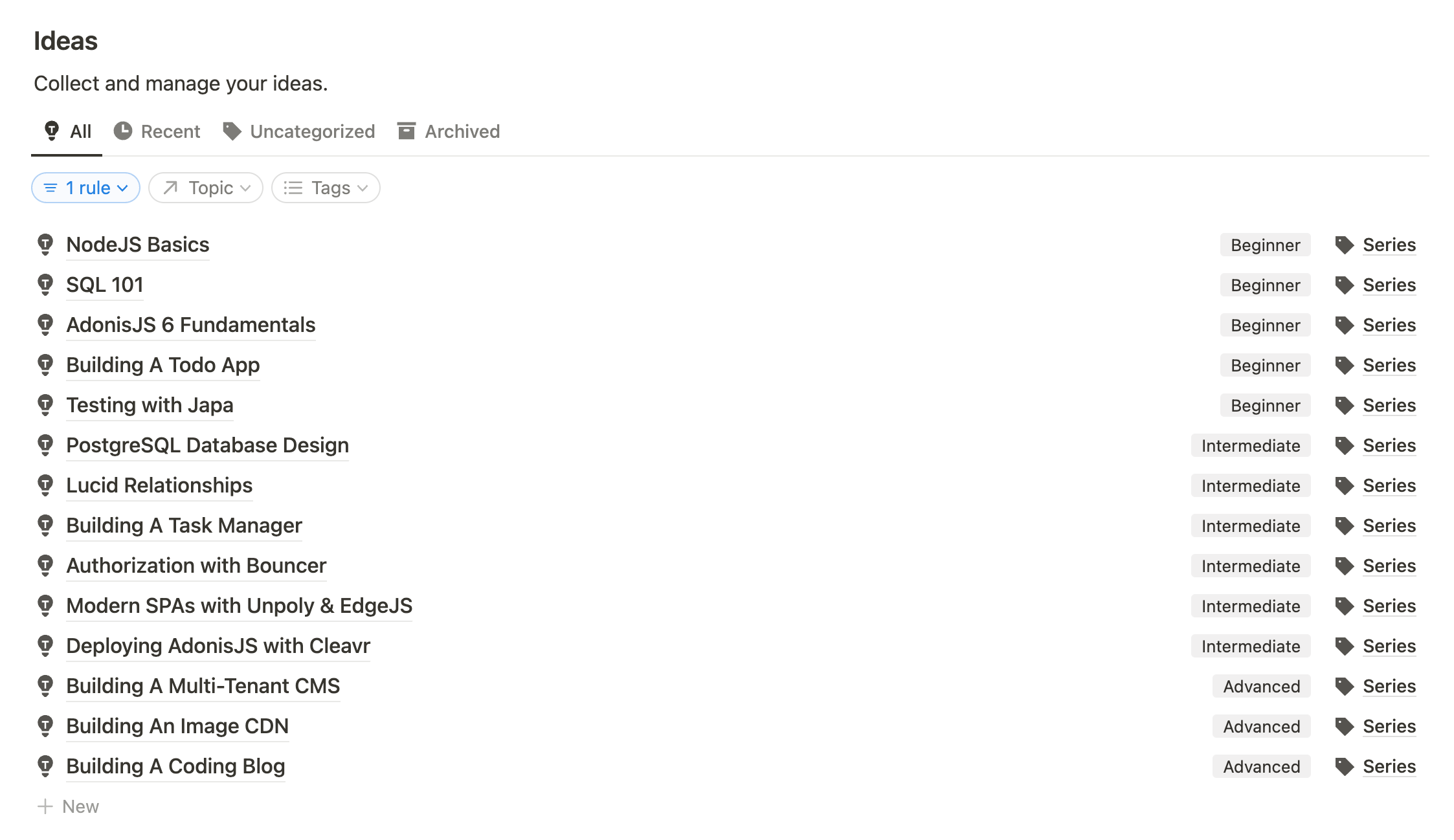The image displays a plain white page featuring black text. At the top, the heading reads "Ideas." Accompanying this title is a motivational subtitle, "Collect and manage your ideas." Below the heading, there are four categories listed: All, Recent, Uncategorized, and Archived, each represented by a distinct symbol. Next to the "All" category, there appears to be a symbol resembling a light bulb containing the letter 'T' inside it.

Underneath these categories, the text outlines various educational series divided by level of complexity. These include:

- **Beginner Series:**
  - Node.js Basics
  - SQL 101
  - AdonisJS: Six Fundamentals
  - Building a To-Do App
  - Testing with JAPA

- **Intermediate Series:**
  - PostgreSQL Database Design
  - Lucid Relationships
  - Building a Task Manager
  - Authorization with Bouncer
  - Modern SPAs with Unpoly and EdgeJS
  - Deploying AdonisJS with CLEAVR

- **Advanced Series:**
  - Building a Multi-Tenant CMS
  - Building an Image CDN
  - Building a Coding Blog

Beneath this list, there is a plus sign accompanied by the word "New," inviting the user to create a new entry.